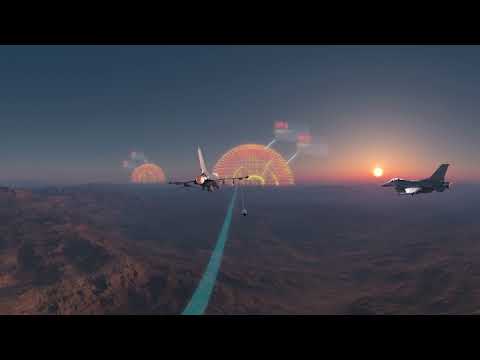The image appears to be a highly realistic screenshot from a flight simulator or video game, depicting two fighter jets in mid-air. The central jet, seen from behind, is flying towards a circular geometric pattern on the horizon, which seems to be a target marked by the game. A faint blue line trails beneath it, suggesting a flight path or targeting system, while a missile seems to be deploying from its right wing. To the right, the second jet is also in motion, heading towards a setting sun. The sky is a gradient of dark blues and the burning hues of sunset, creating a dramatic backdrop. Below, the terrain reveals rugged, rocky, and mountainous regions, adding to the scene's realism. In the distance, blurred sunspot-like bursts in hues of orange and yellow could be reflections or in-game effects related to targeting, contributing to the scene's immersive atmosphere. The overall composition suggests a dynamic scenario, possibly simulating a military exercise or combat mission.